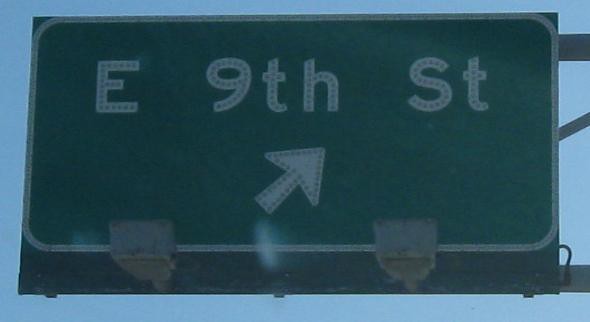An image features a blue sky in the background. Dominating the scene is a street sign with a green label and a white border, prominently displaying the text "East 9th Street" in white, dotted letters. The sign is slightly grainy, indicative of lower image quality. Each letter, including the "E" in "East" and the "9th Street" text, is filled with small metal dots, suggesting they might illuminate or reflect light. There are also directional elements: an arrow pointing to the top right. Additionally, the image includes structural elements, with a horizontal bar extending from the top across to the right, and another bar coming across from the bottom. These details hint at a comprehensive street-sign framework, capturing the essence of an urban environment.